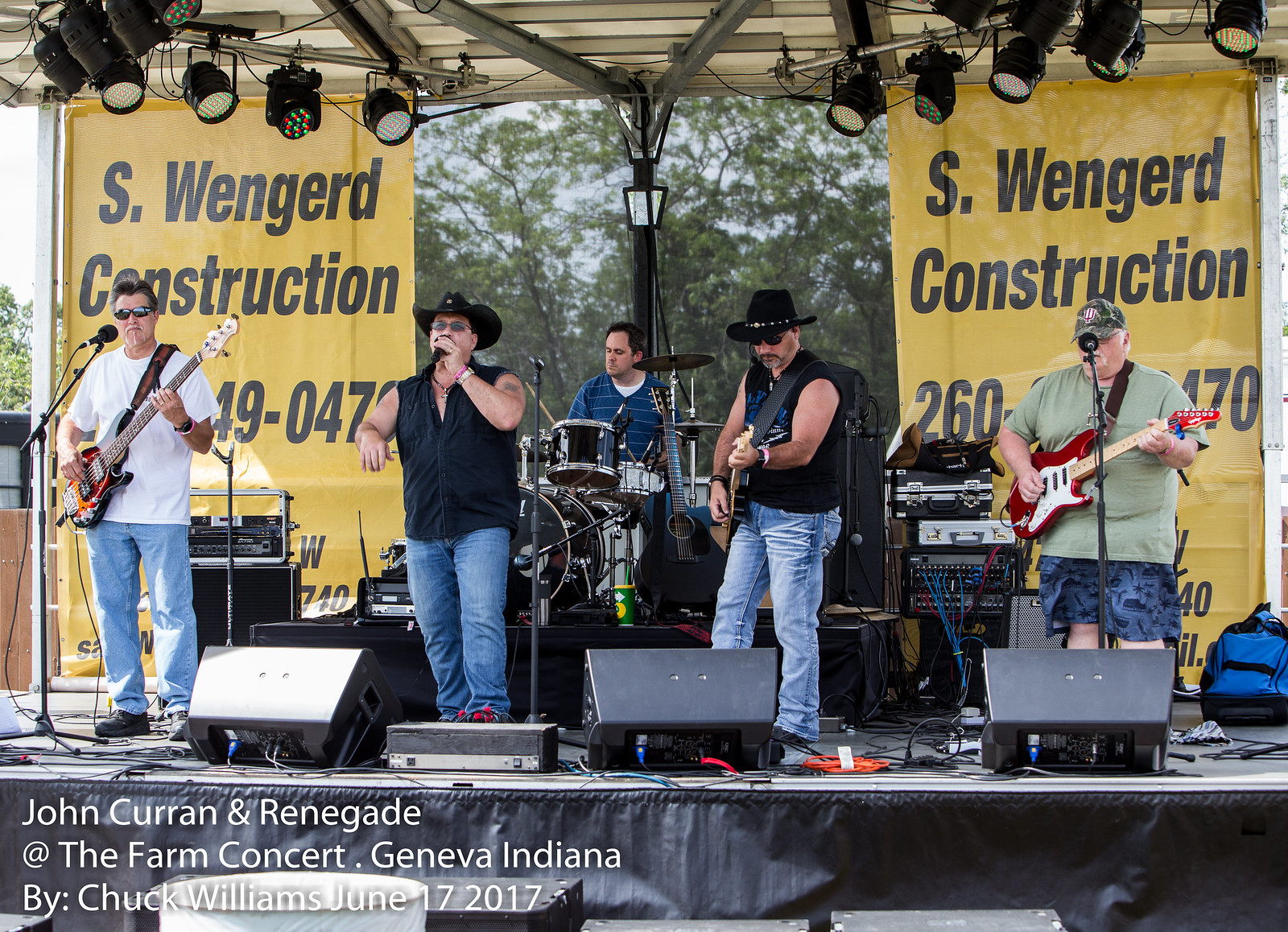In this visually captivating image taken by Chuck Williams on June 17, 2017, during the "At the Farm Concert" in Geneva, Indiana, we see a vibrant outdoor band performance. The stage features five members of the band "John Curran and Renegade." On the far left, a guitarist dressed in a white t-shirt and blue jeans plays confidently, partly obscuring the phone number on the tall yellow banner behind him. The banner, clearly advertising "S. Wengerd Construction," is also mirrored on the right side of the stage.

From left to right, the band members include a singer with a black cowboy hat, black sleeveless button-down shirt, and blue jeans, holding a microphone up to his face. Next to him, another guitarist, also in a black cowboy hat and sleeveless t-shirt, matches the casual yet coordinated stage attire. Further to the right, a larger man in a camo baseball cap and light green shirt with blue shorts strums his guitar passionately. Behind these musicians, the drummer, wearing a blue striped shirt over a t-shirt, is perched on an elevated platform, adding rhythm to the ensemble.

Above the stage, stage lights complete the setup, while the prominent yellow banners bearing the "S. Wengerd Construction" name frame the performance area. The bottom-left corner of the photo includes a white watermark noting the event, the band name, and the photographer's credit: "John Curran and Renegade at the Farm Concert, Geneva, Indiana by Chuck Williams, June 17, 2017."